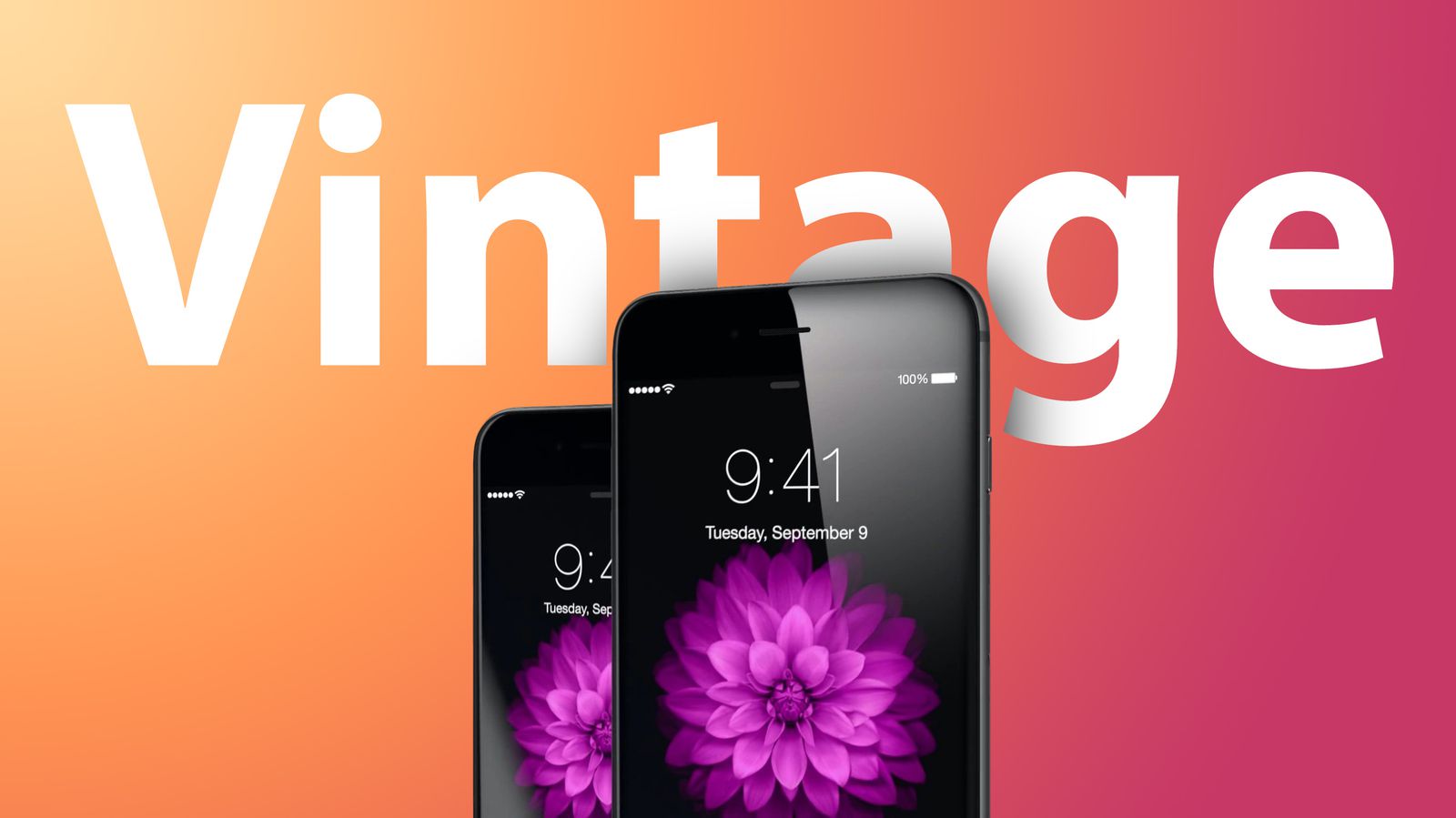In this vibrant advertisement, two identical black iPhones, both displaying the time 9:41 and date Tuesday, September 9th, are prominently featured. Their screens showcase the default iPhone background of a detailed purple flower with numerous tiny petals. The devices are fully charged at 100% and show full Wi-Fi signal strength. These iPhones are slightly staggered, with one positioned slightly higher and to the right of the other, casting shadows on the backdrop. The background of the image features a striking gradient transitioning from bright orange to hot pink. Behind the iPhones, the word "VINTAGE" stands out in white block letters, although the letters "T" and "A" are partially obscured by the phones.